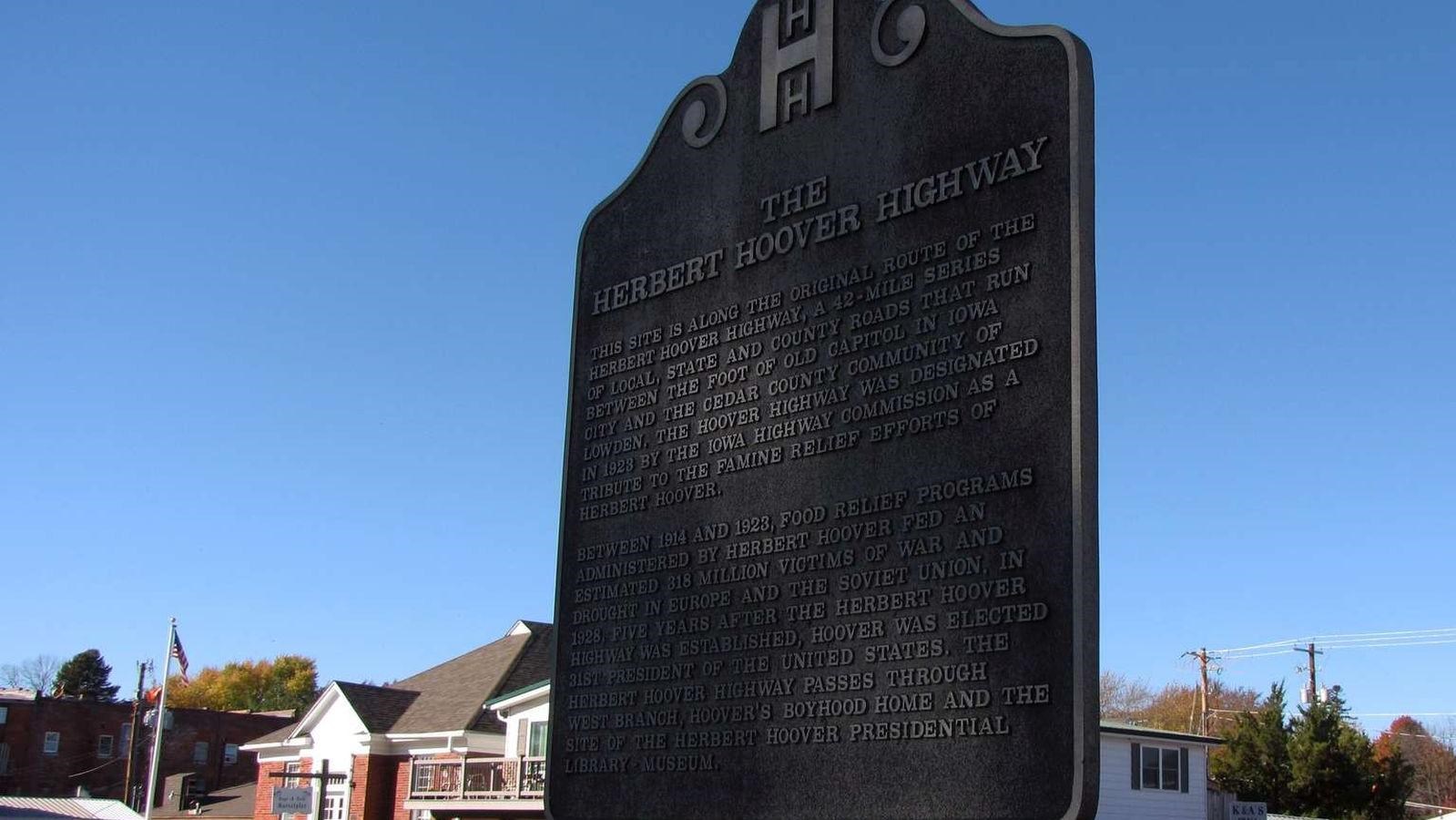This image features a close-up of a black memorial plaque dedicated to the Herbert Hoover Highway, prominently positioned at the center of the frame. The plaque, which has a distinctive tombstone shape, is adorned with a double H logo at the very top followed by text that describes the significance of the highway. The Herbert Hoover Highway, established in 1923 by the Iowa Highway Commission, is a 42-mile stretch that connects the Old Capitol in Iowa City to the Cedar County community of Loudoun. It honors Herbert Hoover's significant famine relief efforts in Europe and the Soviet Union between 1914 and 1923, where he helped feed an estimated 318 million people. Notably, the highway passes through West Branch, Hoover's boyhood home, and the site of the Herbert Hoover Presidential Library Museum. In the background, one can discern a small red-brick building with what seems to be a deck and chairs, a hanging sign, and various trees. An American flag flutters from a flagpole on the left side of the image, while power lines and telephone poles are visible on the right, all set against a clear blue sky.